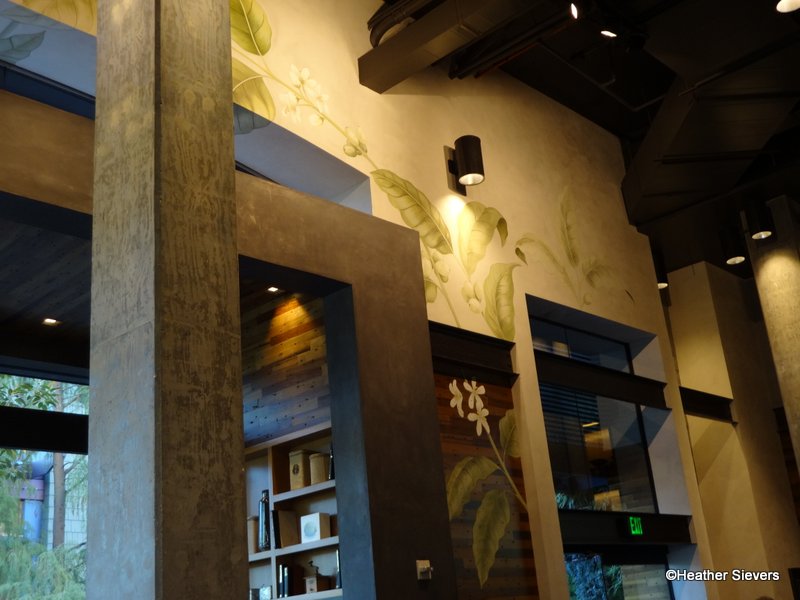This slightly blurry large square photo captures the interior of a building, taken at a slightly upward angle. The walls, painted a muted golden-brown color, feature a delicate pattern of green leaves and small white flowers. A cylindrical black light fixture shines down from near the top of the picture, illuminating part of the leafy design. In the lower right corner, a copyright symbol and the name "Heather Seavers" (S-I-E-V-E-R-S) in white text can be seen.

On the left side of the image, a prominent wooden column extends from the bottom to the top of the frame. Adjacent to this column, a wooden casing forms an entranceway to another room. The entryway has visible wooden shelves lined with various objects, and further left, in the corner, a window reveals a glimpse of trees or buildings outside. The upper part of the wall showcases the detailed leafy pattern, accentuated by the lighting, while the right side remains plain without the decorative vines. The left side also shows part of the ceiling with lights installed, contributing to the warm ambiance of this apparently evening scene.